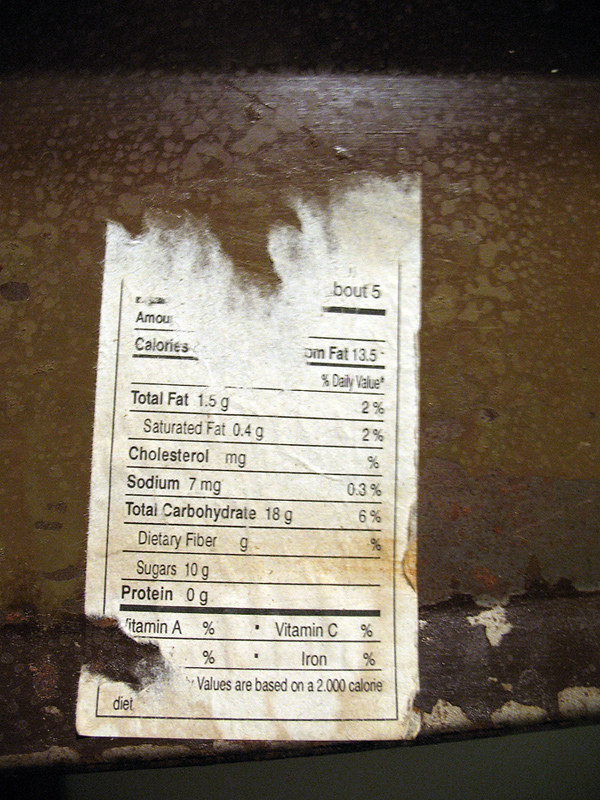The image features a heavily rusted metallic object with an old, tattered nutritional facts sticker adhered to its surface. The rust is so severe that it has corroded the metal and invaded the sticker itself, rendering it partially illegible. The top half of the sticker is almost completely worn away, while parts of the bottom left are also missing. What remains legible on the sticker includes nutritional details like "total fat 1.5g (2%)," "saturated fat 0.4g (2%)," "cholesterol," "sodium 7mg (0.3%)," "total carbohydrate 18g (6%)," "dietary fiber," "sugars 10g," "protein 0g," and percentages for vitamins A, C, and iron. The label seems to originate from a food product but now resides on an unidentifiable, deteriorating surface, giving the entire scene a decrepit, abandoned look.